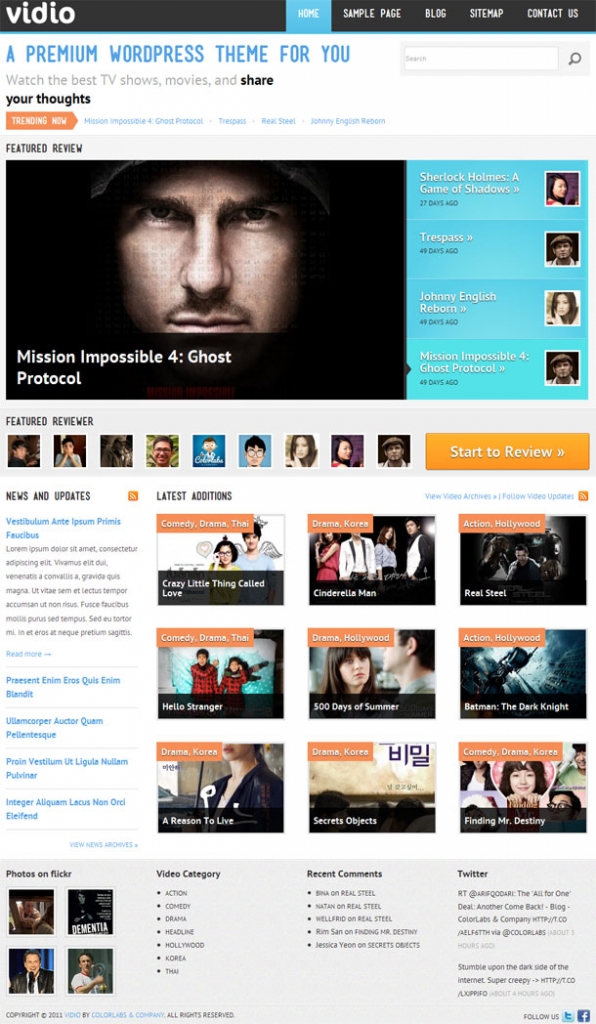The image is from the website "Video" (spelled as V-I-D-I-O), featuring a sleek black banner at the top that prominently displays the brand name. The banner includes several navigation tabs for easy browsing: Home, Sample Free, Blog, Site Map, and Contact Us. Below the banner, blue text reads "A premium WordPress theme for you," accompanied by a search bar designed to help users narrow down their search.

Beneath this section, the tagline "Watch the best TV shows, movies, and share your thoughts" sets the tone for the site’s offering. Highlighted below is a "Feature Preview" section showcasing the movie "Mission Impossible 4: Ghost Protocol." The focal point of this area is an image of a Caucasian male character set against a dark background, giving an intense look at the viewer. Next to this visual, a blue banner provides a brief description, likely outlining the characters in the movie.

Further down, the "Featured Reviewers" section displays a series of square boxes, each containing the image of different individuals. Adjacent to each image is a small orange banner that invites users to "Start to Review," offering the option to watch and review their movie of choice.